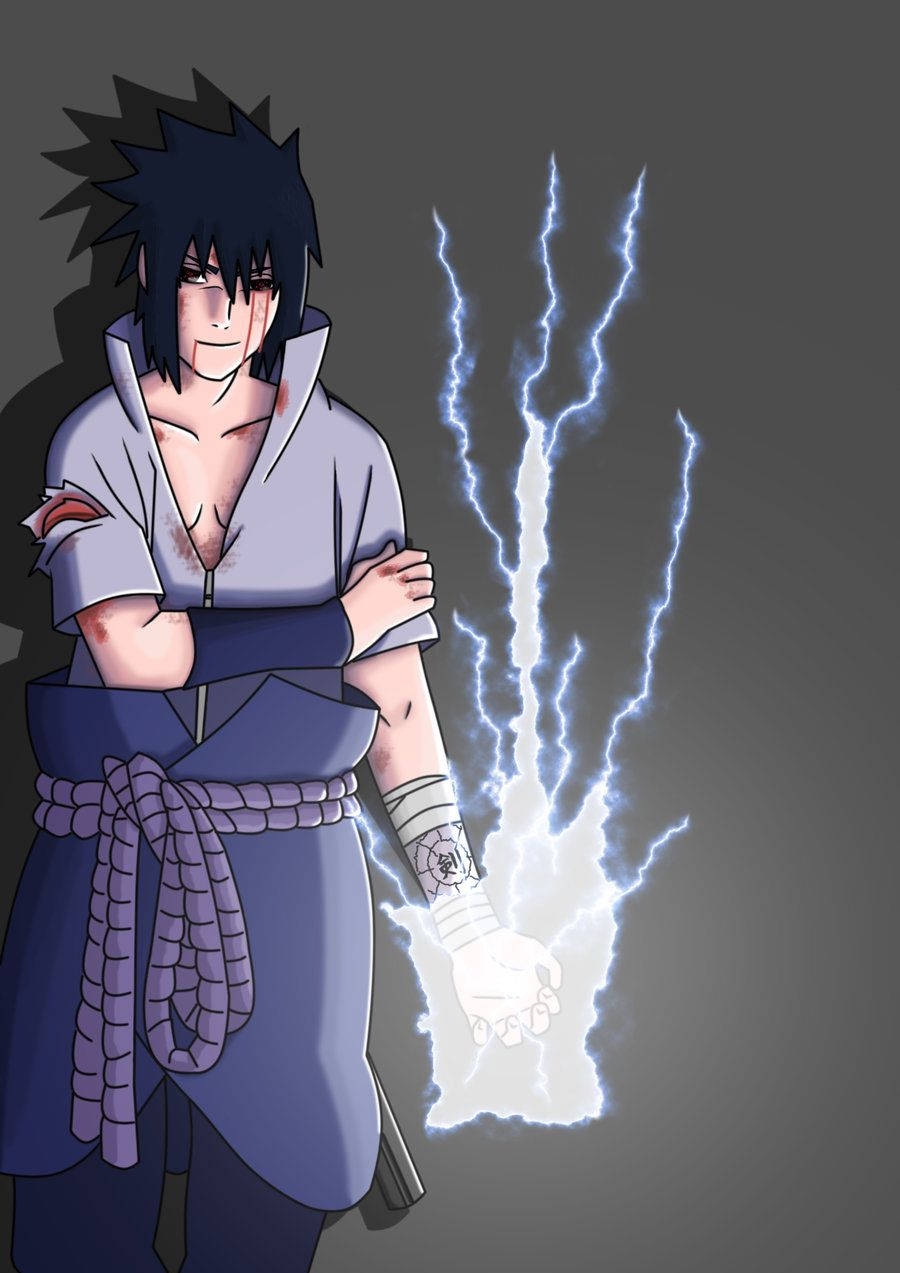The image depicts an anime-style character standing on the left side of the frame. He has short, spiky black hair with longer strands framing his angular face, marked by black, angular eyes. He is dressed in a gray collared shirt that opens at the chest, revealing part of his pectoral muscles, with the collar extending up to his ears. His clothes show signs of battle, with scratches, bruises, and blood. There is a notable tear in his shirt and a cut on his left arm, which also features a geometric tattoo. He wears a black arm guard on his forearm and dark blue pants, secured with a large rope, with a light blue cloth overlay. His right arm is draped over his left, while bolts of lightning emanate from the palm of his left hand. Despite his injuries, he faces the camera with a resilient smile.